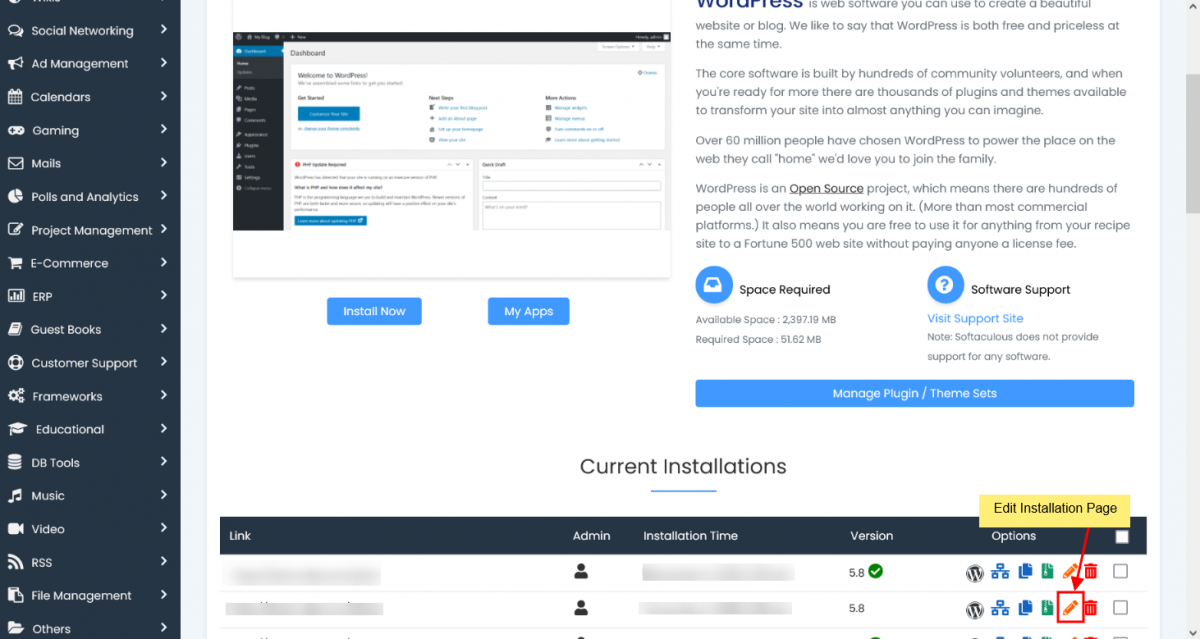This image captures a partial screenshot of a WordPress dashboard, showcasing the user interface and navigation elements. The main vertical menu on the left side of the webpage features a dark charcoal background with white text and includes options like Social Networking, Ad Management, Calendars, Gaming, Mails, Polls, and Analytics. 

In the central part of the image, a smaller rectangle displays the dashboard's welcome message, "Welcome to WordPress," although it appears blurry. Further to the right, a cut-off section highlights the word "WordPress" in dark blue. This section begins with a description: "WordPress is web software you can use to create a beautiful website or blog," but much of the text is incomplete.

Towards the bottom of the image, the partially underlined, centered text "Current Installations" is prominently displayed in blue. Below this, another dark tab with white lettering lists columns for Link, Admin, Installation Time, Version, and Options. A yellow rectangle labeled "Edit Installation Page" is accented by a red arrow pointing to a red pencil icon enclosed in a red square box, drawing attention to the function for editing the installation page.